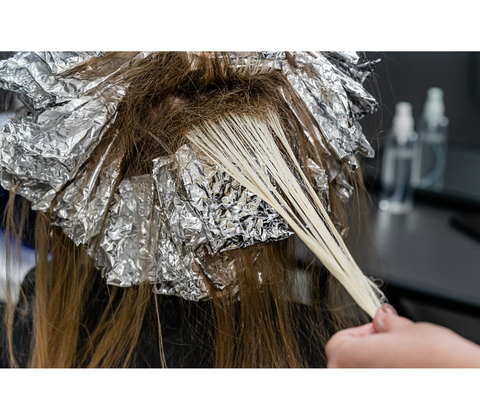In the image, a woman with long, brunette hair is seated in a salon chair, undergoing a bleaching treatment. Her hair is sectioned and wrapped in numerous crumpled squares of silver aluminum foil, which cover roughly 75-80% of the photo's frame. A single left hand, adorned with painted nails, is in the process of handling a platinum blonde strand, either checking its progress or beginning to remove the foil. The salon setting is indicated by the background, where a clear spray bottle with a white atomizer top sits on a grayish-black counter, partially reflected in a nearby mirror. The focus remains tightly on the woman’s hair and the bleaching process, highlighting the intricate details and method commonly used in hair treatments.